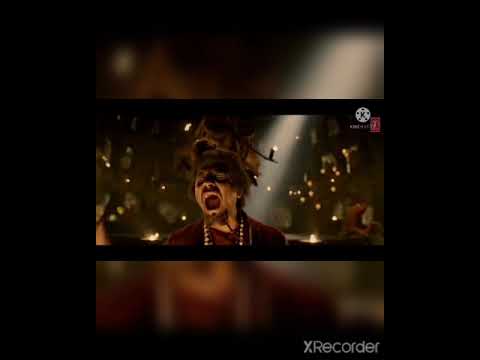This image is a screenshot from a video player, featuring a vivid portrayal of a man screaming in apparent agony. Central to the composition is a close-up of the man, who has brown, unruly hair piled on top of his head and a distinct beard that is split into two braids. His eyes appear gouged out, enhancing the intensity of his open-mouthed scream. He wears a maroon top and a necklace around his neck, adding to his distinctive appearance. The background is dimly lit, with a dotted pattern of yellow lights or candles and a prominent shaft of white light streaming down from the top right corner. This central image is flanked by black vertical bars on either side, and there is an overlaid, blurry close-up at the top and bottom sections, focusing on his shoulders and head. The entire image is framed by a black rectangle, with the word "X recorder" displayed at the bottom center, indicating the use of a screen recording app.